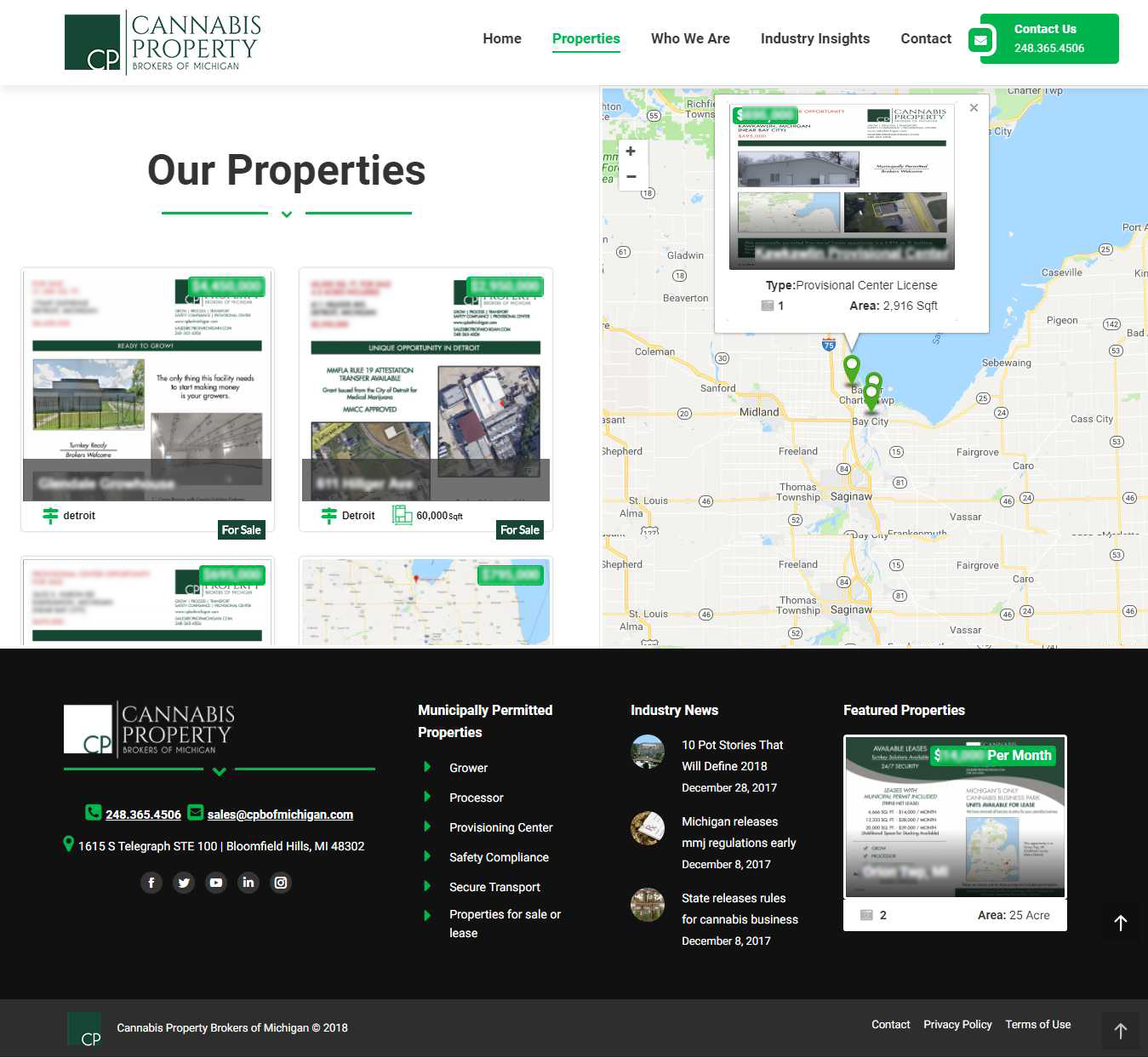Screenshot of the Cannabis Property Brokers of Michigan website. In the upper left corner, the website logo prominently displays "Cannabis Property Brokers of Michigan." To the right, navigational buttons include "Home," which is currently selected and underlined in green, "Properties," "Who We Are," "Industry Insights," and "Contact." Below this menu, a green rectangle features the text "Contact Us" followed by the phone number (248) 365-4506.

The main section titled "Our Properties" showcases listings, though the information is blurred out. On the right side of the page, there is a map with three marked drop points indicating property locations.

At the bottom, contact information is provided: phone number, email address (sales@cpbofmichigan.com), and various section headings including "Industry News," "Featured Properties," "Municipally Permitted Properties," "Contact," "Privacy Policy," and "Terms of Use."